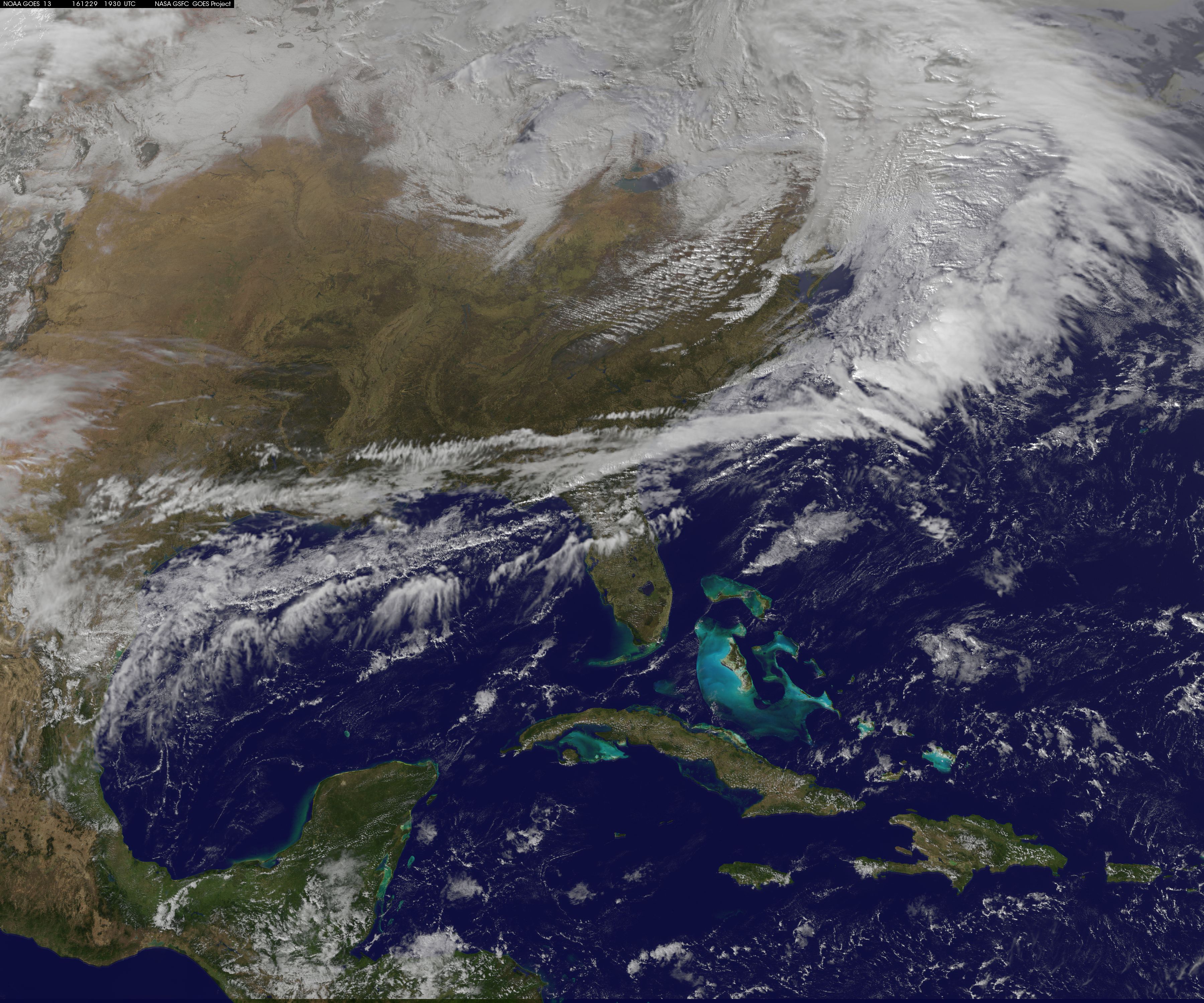A high-resolution satellite image taken from space showcases the eastern part of the United States and the Gulf of Mexico. The deep blue oceans starkly contrast with the lighter blue shallows surrounding various islands, including the Florida Keys and Cuba. The green terrain of the United States, Mexico, and Cuba transitions from lighter to darker olive shades, indicating varying landscapes and mountain ranges. Distinct cloud formations hover over the land and water, with a significant storm system visible over the Gulf of Mexico. This system features a beige inner area surrounded by extensive swirling white clouds. In the bottom left-hand corner, you can make out part of Central America. The image also depicts the diverse colors of the terrain, from green islands to brown swirls indicating mountainous regions, giving a comprehensive view of this part of the Earth from space.